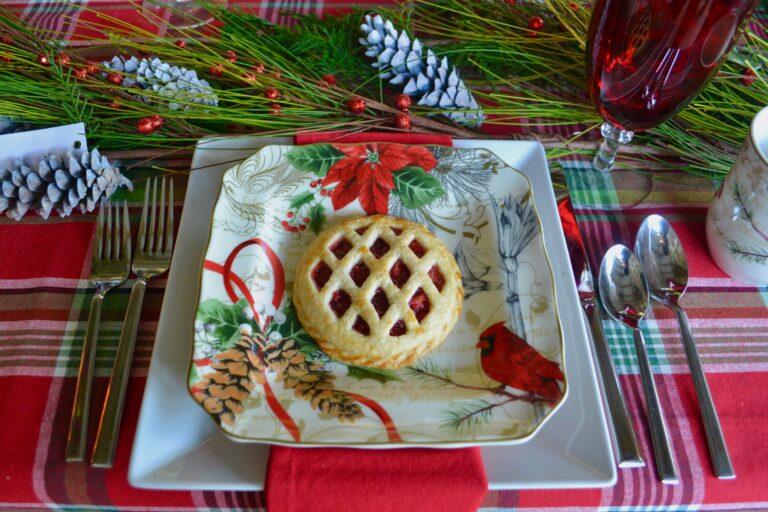The image features an elegantly set table with a Christmas theme, centered around a delectable small cherry pie with a lattice top. The pie rests on a beautifully decorated plate adorned with pinecones, greenery, red ribbons, and a cardinal perched on a branch. This decorative plate is placed on top of a larger plain white plate, creating a layered effect. The table setting includes a red plaid tablecloth, enhancing the festive feel. Surrounding the plate, there are utensils meticulously arranged: two forks to the left, two spoons and a knife to the right, along with a vibrant red stemware glass. Additional holiday elements such as pinecones dusted with white, sprigs of greenery, and red holly berries are scattered artfully across the tablecloth. A neatly folded red napkin sits to the right, complementing the overall color scheme and adding a final touch of elegance to the holiday setting.